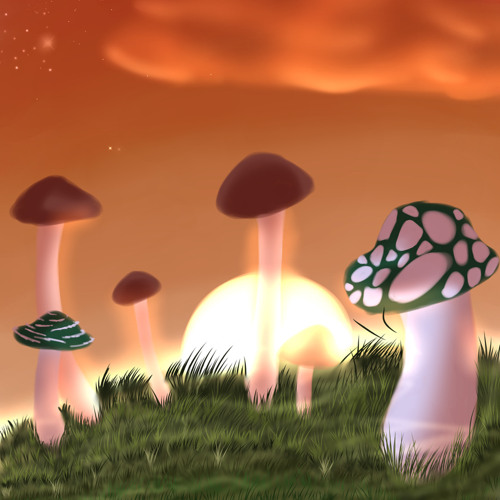This computer-generated fantasy art image features a vibrant and whimsical scene dominated by a variety of mushrooms of different heights, thicknesses, and designs. Set against a striking orange sky tinged with touches of brown, the atmosphere evokes an enchanting sunset with a large, white cloud and several stars scattered in the top left corner. The grassy field appears almost cartoon-like with exaggerated green blades.

In the foreground, two green mushrooms steal attention. The larger one, positioned centrally, boasts large white spots, while the smaller one on the left side is adorned with bright white stripes. Further back on the left side, three mushrooms with red caps stand tall, alongside a shorter mushroom with a white cap.

Each mushroom is connected by uniformly pink stems of varying thickness. One notable mushroom, located towards the back with a thick stem, features a green and pink cap adorned with pink polka dots. Another mushroom displays a green and white cap with white lines.

This childlike artwork is characterized by its imaginative use of color and playful design, providing a glimpse into a fantastical world where even the sky itself adds to the dreamlike quality of the scene.